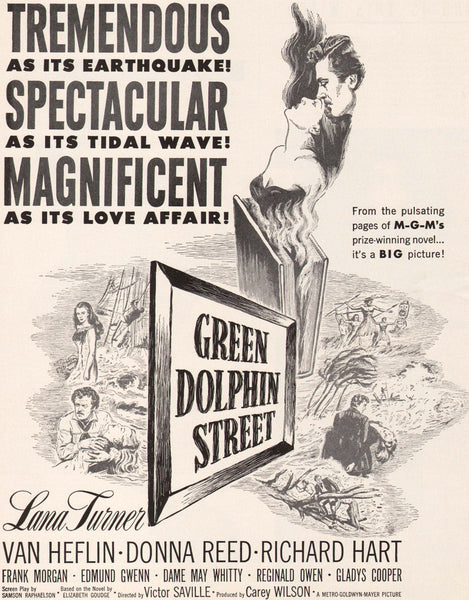This black-and-white, hand-drawn movie poster, professionally crafted for MGM's prize-winning novel adaptation "Green Dolphin Street," is striking with its vivid imagery and dramatic text. At the top left, bold black text exclaims, “TREMENDOUS as its EARTHQUAKE! SPECTACULAR as its TIDAL WAVE! MAGNIFICENT as its LOVE AFFAIR!” In the center, a stunning illustration captures attention: a woman in a low-cut, sleeveless bustier with long black hair, leans back as a man intimately kisses her forehead. She appears to be emerging from an open book. Surrounding this central image are smaller scenes in grayscale, depicting various characters and moments from the film, including a woman possibly dancing, another woman passed out in a man's arms, a serious-looking man in a suit, and a solemn-looking woman standing alone. Below this collage, a framed sign announces “Green Dolphin Street.” The bottom section prominently features the names of the starring actors: Lana Turner, Van Heflin, Donna Reed, Richard Hart, Frank Morgan, Edmund Gwenn, Dame May Whitty, Reginald Owen, Gladys Cooper, Victor Saville, and Carrie Wilson.